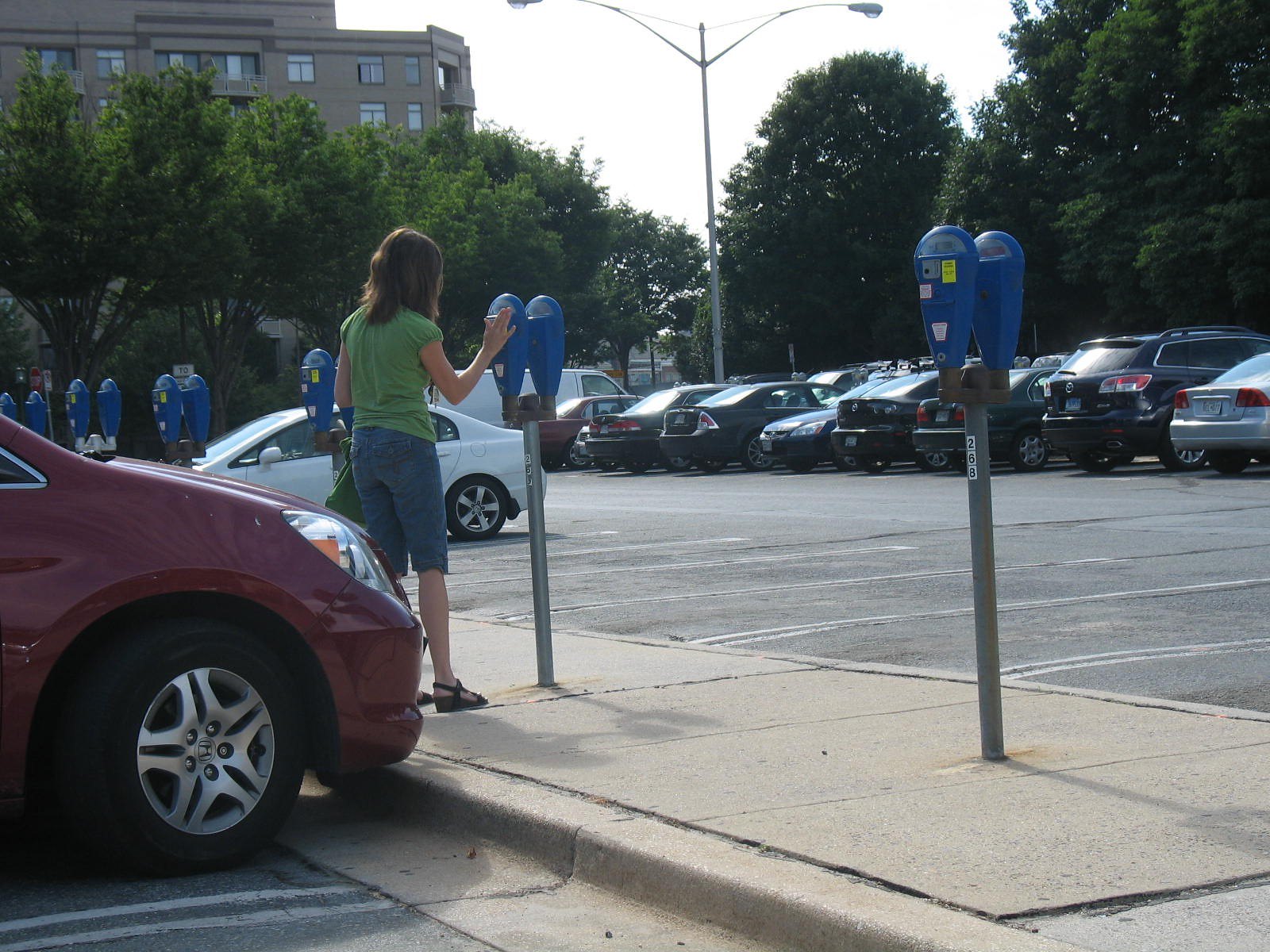This color landscape image captures a bustling parking lot taken from the perspective of someone sitting in their car. The focus is on a series of blue parking meters mounted on weathered metal poles, which are lined up along a raised sidewalk-like median. The meter line progresses from right to left as it recedes into the distance. Of particular note, a woman stands at the second meter from the camera, wearing a green cap sleeve shirt, denim cut-off shorts, and strapped sandals akin to Tevas. She has long brown hair that drapes just past her shoulders. Her car, a dark red or burgundy SUV, is positioned to the right, and she appears to be paying the parking fee. The lot contains mid-2010s era vehicles, one of which is adjacent to the raised curb on the far side. The image is underlaid with the greenery of trees that line the parking area, with the upper left of the image revealing a multi-story building behind the foliage. Street lamps are visible at the top center of the frame, adding urban context to the serene scene.